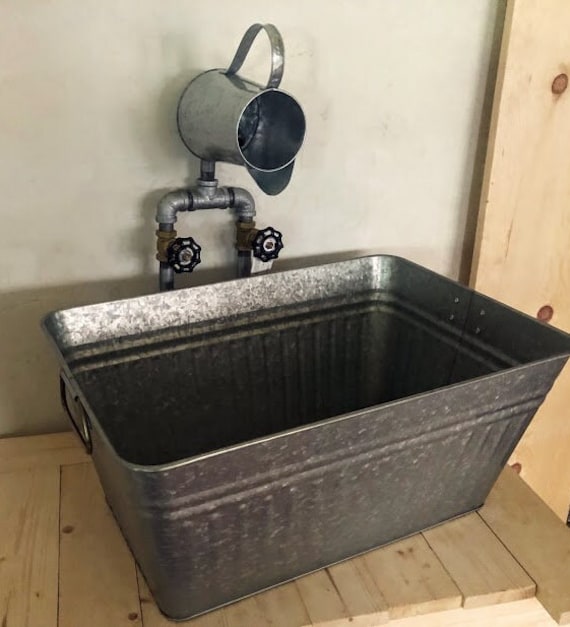The photograph showcases an old-fashioned, antique washtub made of a lightweight metal, likely aluminum, with a rectangular shape measuring approximately three feet in length, two and a half feet in width, and 16 to 18 inches in height. The washtub, resembling a large laundry basket, features two handles on its sides with visible rivets. It rests on a wooden table adorned with beige wood panels accented by thoroughly darkened brown knots. Immediately above the washtub, a silver faucet with two knobs for hot and cold water is attached to a silver metal pole, controlling the flow of water into the basin. Additionally, a large, metal antique camp cup or pitcher hangs over the washtub. Behind the setup is a green ball placed against a black metal container, leaning against the wall. The overall scene evokes a vintage, rustic feel, harmonizing the elements of wood, metal, and aged craftsmanship.